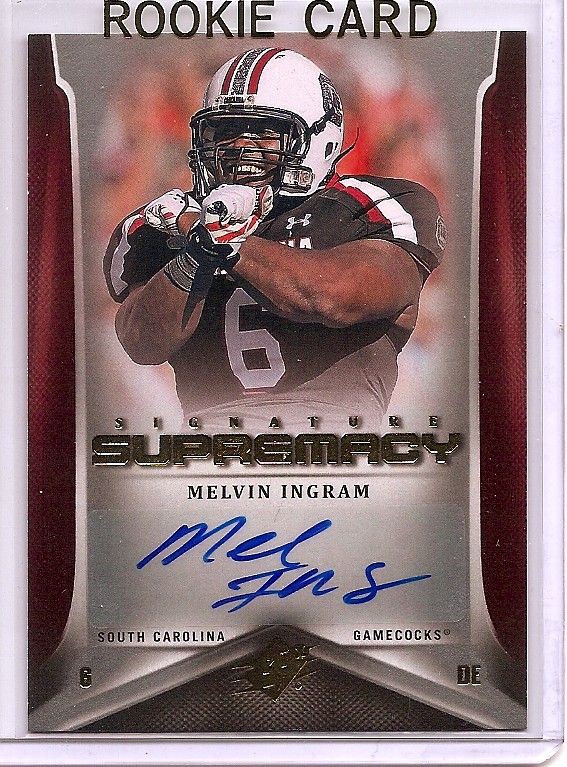This is a detailed description of a football rookie card featuring Melvin Ingram. The card is encased in a protective glass case and prominently labeled "Rookie Card" at the top. The card showcases a picture of Melvin Ingram in his football uniform. He is wearing a black jersey with red and white stripes on the shoulders, featuring the number six in white. Above his chest, his arms are crossed in an X formation while he smiles, wearing a white helmet with red and silver stripes. Beneath his picture, the card reads "Signature Supremacy Melvin Ingram" and includes his autograph in blue Sharpie, with the inscription "Mel Ingram." Additionally, the card denotes his college team, the South Carolina Gamecocks, and features the initials "C" in the bottom left corner and "DE" in the bottom right corner, likely indicating his position.